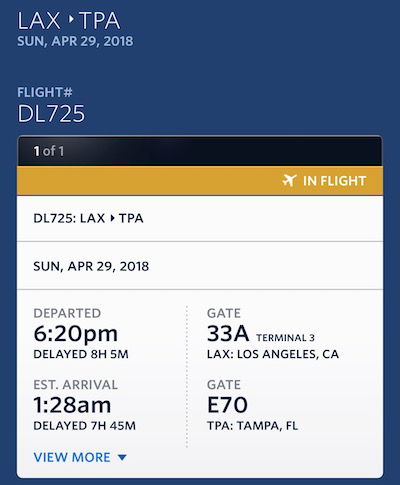This image is a detailed flight information display featuring a predominantly blue box design with a central white square. At the very top, "LAX" is prominently displayed with a small white arrow pointing to "TPA," indicating the flight is bound for Tampa, Florida. The date "Sunday, April 29th, 2018" is also included at the top. Below this, the flight number "DL725" is clearly written in white capital letters within the square. 

On the right side of this central section, a small black bar prominently shows the number "101," and directly below, a gold bar features the word "in-flight" along with a small airplane icon. Beneath this, on a purely white background, the flight details are reiterated with "DL725" from "LAX" (Los Angeles International Airport) to "TPA" (Tampa International Airport). The following line includes the date "Sunday, April 29th, 2018."

Further information reveals that the flight "departed at 6:20 p.m." but was delayed by "8 hours and 5 minutes," with an "estimated arrival" now at "1:28 a.m." Below this, another updated delay of "7 hours and 45 minutes" is noted. At the bottom, there is a link with blue text stating "view more" accompanied by a small arrow.

On the right-hand side of the white square section, the gate information is detailed. The departure gate from LAX is listed as "Gate 33A, Terminal 3," and the arrival gate at TPA (Tampa, Florida) is mentioned as "Gate E70."